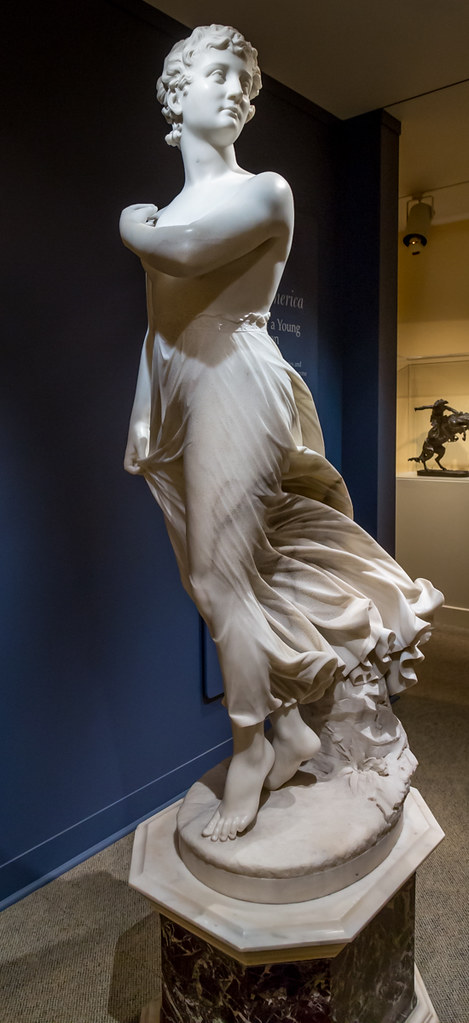This photograph captures a stunning, life-sized marble statue of a woman set against a museum backdrop. The main figure stands gracefully, with her right arm down at her side, gently pulling on her flowing skirt, and her left arm raised to touch her right shoulder. Her head is elegantly turned to her left. The artist has rendered the marble with such skill that the gown appears to be flowing, giving a sense of movement. 

The statue stands atop a detailed pedestal that combines lighter and darker shades of stone, possibly a mix of marble and granite. The background features a blue wall adorned with some white writing, of which the word "young" is discernible. Additionally, another display case showcases a smaller Western-style statue of a cowboy riding a rearing horse. 

Illuminated by a track light, the main focus of the photograph—the exquisite Greek-inspired marble statue—commands attention within the museum setting, showcasing the artist's incredible craftsmanship and attention to detail.